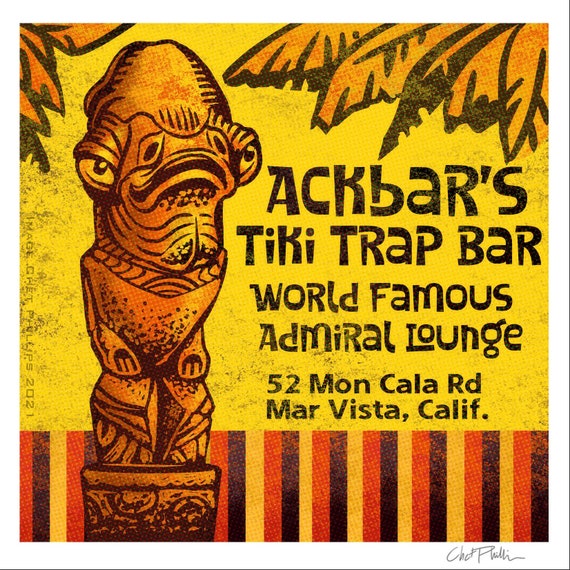This is an advertisement poster for Ackbar's Tiki Trap Bar, designed to resemble a square flyer. The background is predominantly yellow, with the bottom section adorned with vertical stripes in alternating black, red, dark purple, and yellow colors. On the left side of the flyer, there is a depiction of a tiki statue designed to look like Admiral Ackbar from Star Wars. The statue is orange, with wide-set eyes on the sides of its head, giving it an alien-like appearance, and it stands on a totem. Above and to the sides of the statue, there are brownish-orange palm fronds. In the yellow middle section of the flyer, black text reads: "Ackbar's Tiki Trap Bar - World Famous Admiral Lounge." Below this, the address is provided: "52 Mon Cala Road, Mar Vista, California." At the bottom of the flyer, there appears to be an autograph from someone named Chet Feather.